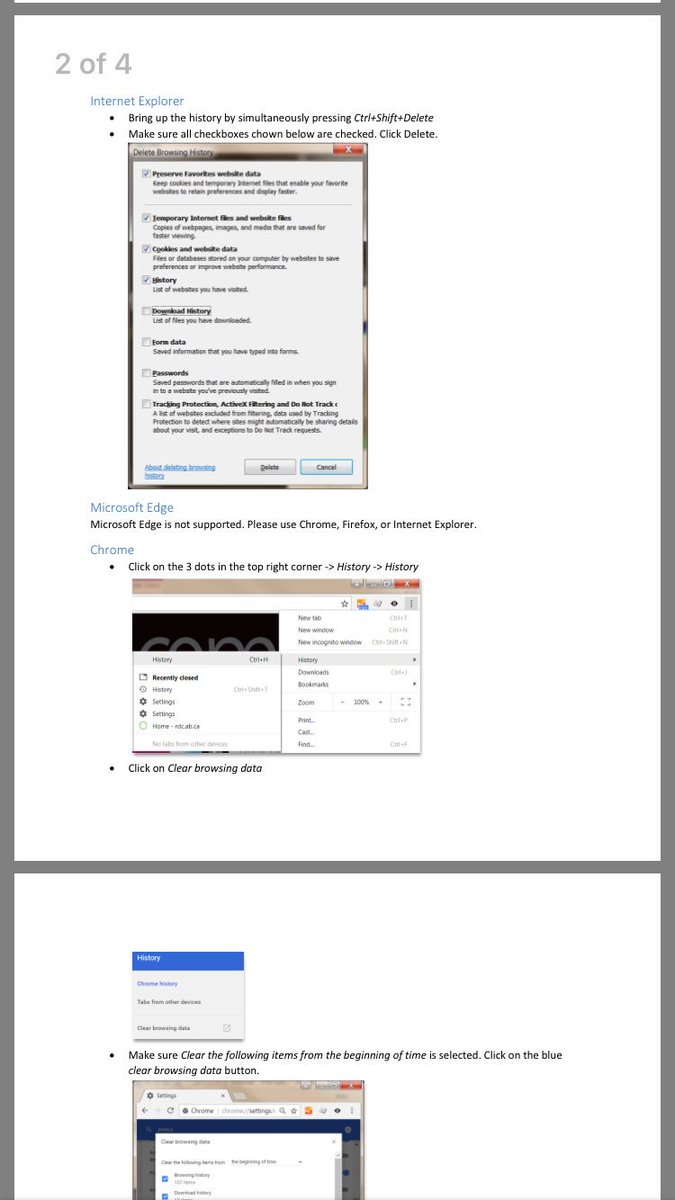**Detailed Image Description:**

The image is a screenshot of a website with instructions on how to clear browsing history for different browsers. The overall layout consists of a gray border surrounding the image, with the content divided into two sections by a green line.

**Top Section:**

- **Background and Text**: The top section has a white background with "Two" written in gray font at the top. Below it, "Internet Explorer" is prominently displayed in blue.
- **Instructions for Internet Explorer**:
  - A bulleted list outlines the steps:
    - "Bring up the history by simultaneously pressing Control + Shift + Delete."
    - "Ensure all checkboxes shown below are checked."
    - "Click Delete."
  - Accompanying this text is an image of a Windows dialog box titled "Delete Browsing History," highlighting the "Delete" button.

- **Microsoft Edge**:
  - A statement in this section indicates that "Microsoft Edge is not supported. Please use Chrome, Firefox, or Internet Explorer."

- **Instructions for Chrome**:
  - Users are instructed to "click on the three dots in the top right corner." An arrow diagram points to "History," followed by another arrow pointing to "History" again, representing the submenu selections.
  - Another bullet point instructs: "Click on Clear Browsing Data."

**Bottom Section:**

- **Background and Text**: This section also has a white background and starts with the word "History" in blue.
- **Further Instructions for Chrome**:
  - "Chrome History" is followed by an illustration or mention of "Clear Browser Data."
  - The final bullet point specifies: "Make sure 'Clear the following items from the beginning of time' is selected."
  - Users are guided to "click on the blue Clear Browsing Data button" to finalize the process.

This comprehensive breakdown in the image provides step-by-step guidance for clearing browsing data in Internet Explorer and Chrome, mentioning that Microsoft Edge is not supported, with visual aids to help users easily follow the instructions.